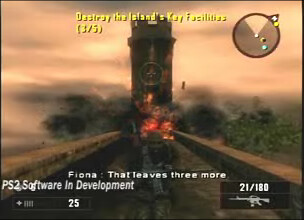The image depicts a blurry, low-resolution screenshot of a video game. It is a square image bordered in black, with the top of the screen displaying a yellow text directive: "Destroy the island's key facilities (3/5)." Below a pink and gray sky, an armored soldier character runs toward the foreground on a brown bridge. In the backdrop, an imposing dark tower looms, partially obscured by an explosion with orange and red flames and smoke. The upper-right corner features a circular in-game map or compass, while the bottom-left corner shows a white number "25" in a rectangle. Additionally, the bottom displays white text reading "Fiona. That leaves three more." Further text states "PS2 software in development." The bottom right corner has a depiction of a machine gun with the ammunition count "21/180."